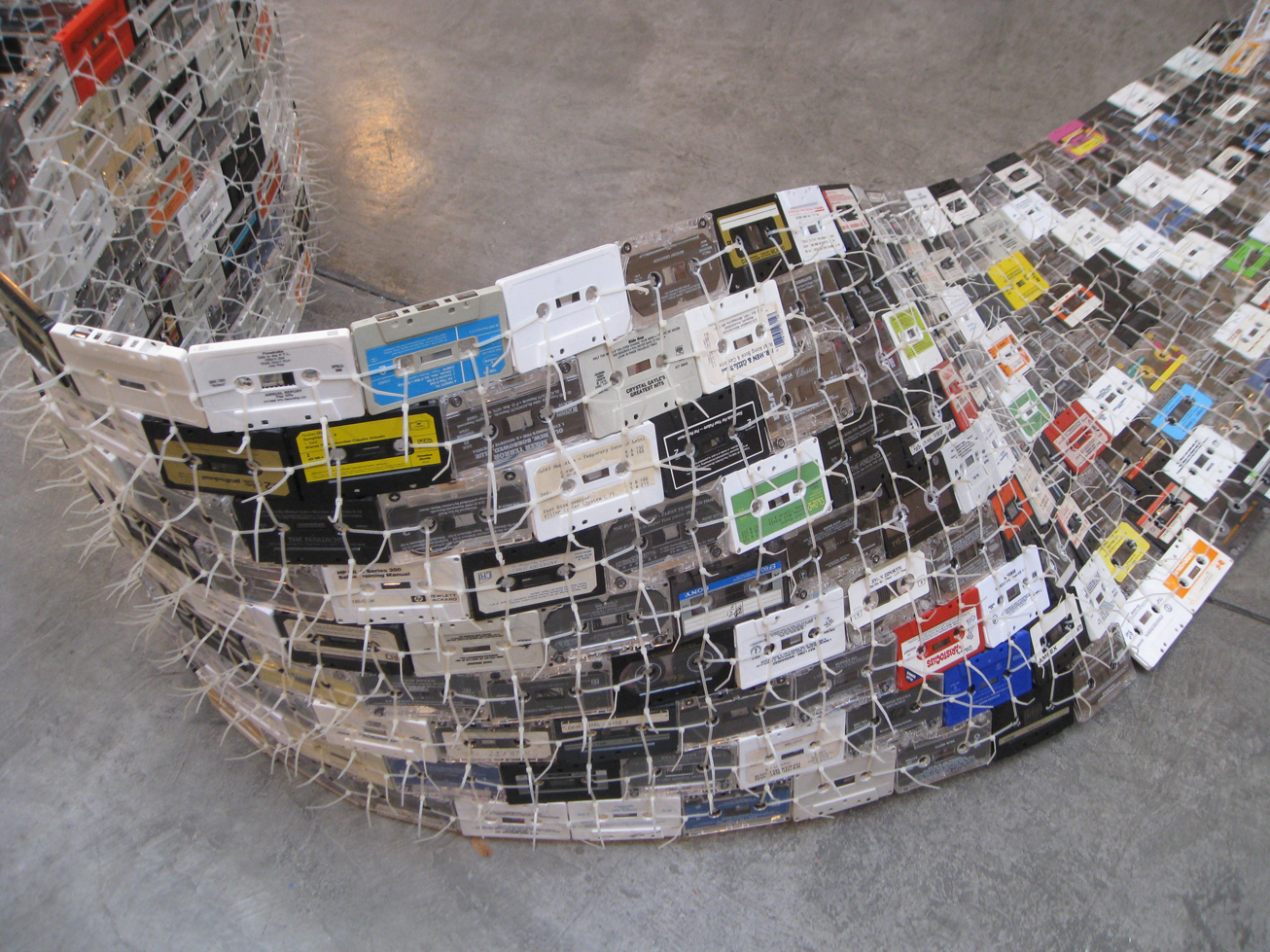The image depicts an intricate art installation composed of a multitude of old cassette tapes. These tapes, in various colors including white, clear, black, red, blue, and yellow, are woven together using zip ties and twist ties to form a fence-like structure on a light gray, stone or concrete floor. The cassette tapes, reminiscent of the 1980s audio era, are arranged in an overlapping brick pattern, with the zip ties connecting their centers to create a cohesive lattice. The installation begins in the top left corner, curves slightly out of frame, then sweeps through the middle before falling flat on the ground and curving back up to the right. The structure appears to be approximately eight to ten tapes high and about two feet wide, extending around 10 to 12 feet in length. Light shadows cast by overhead lamps reveal its complex, ribbon-like form that suggests a flowing, serpentine movement across the floor.